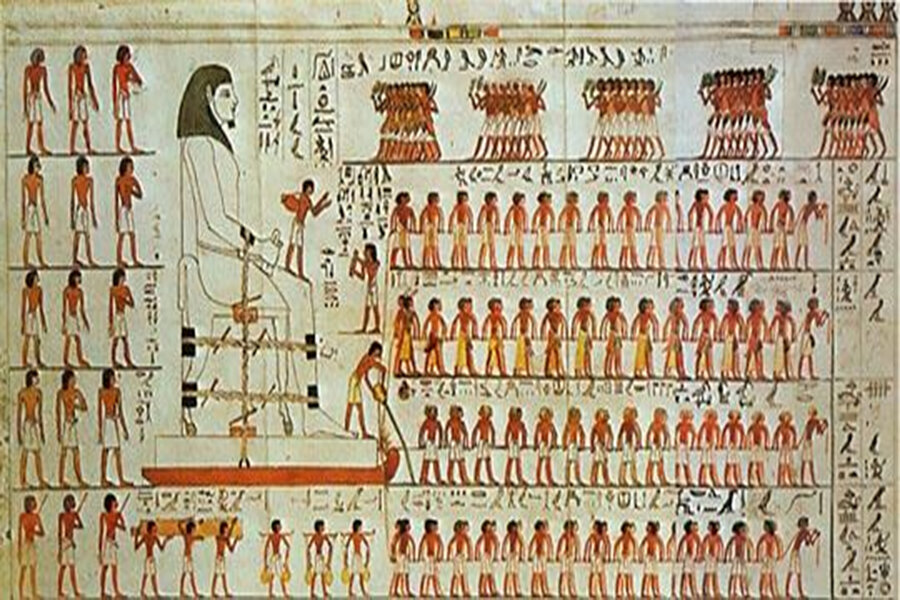The image appears to be a detailed, full-color depiction—either a photograph of a well-preserved ancient Egyptian wall art or a meticulous painting recreating such a scene—of various hieroglyphics and figures. The focus is on multiple rows of shirtless workers clad in white skirts. These individuals are engaged in a coordinated effort, with some using tools or directing the work. The top of the image shows five groups of what appear to be soldiers marching in line. Dominating the scene is a large, possibly carved statue of a pharaoh strapped onto a sled, being moved by the workers. Notably, one person appears to be pouring oil in front of the sled to facilitate its movement. There's also the presence of Egyptian writings, possibly hieroglyphs, and animal images on one side of the artwork. Additionally, a figure, possibly a pharaoh or royal person like a king or queen, is depicted sitting on a throne, with what seems to be a gold chain hanging from their wrist.